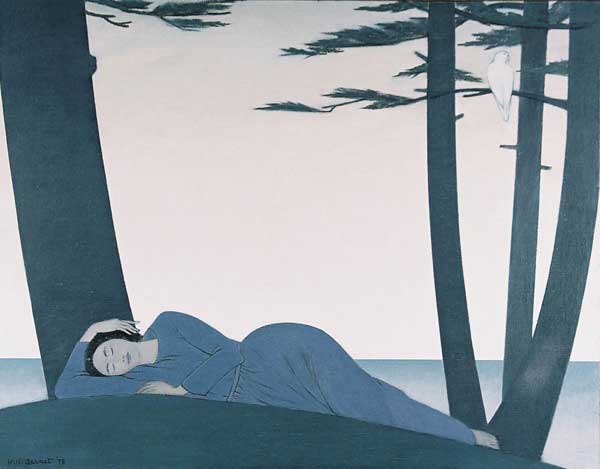The image is a square, cartoonish painting titled "Reclining Woman" by Will Barnett from 1978, featuring a muted color palette dominated by blues, whites, and grays. The sky occupies the entire top half of the painting, presenting a whitish-gray hue. The composition includes landscape elements such as trees and water. On the left side, there is a prominent tree trunk with a few visible branches at the top. Balancing this on the right side are three smaller tree trunks, closer together and adorned with more branches bearing pine needles. A white bird, likely a dove, is perched on one of the branches on the right side, facing away from the viewer.

Centrally, we see a woman lying on a gently sloping hill of blackish-green grass. The ground curves at the bottom edge of the painting. She is dressed in a bluish-gray one-piece outfit or robe tied at the waist. Her long black hair and pale skin suggest she might be of Asian descent, although this is not explicitly clear. She reclines on her right side, appearing to sleep, with her head resting on the upper part of her bent right arm. Her right hand drapes over her left ear, while her left arm extends forward, resting on the ground. Her legs are arranged with one leg bent in front of her.

In the background, behind the woman and the trees, stretches a serene body of water, extending to the horizon. The painting is signed with "Will Barnett '78" in the bottom left corner, adding a final touch of authenticity to this tranquil and introspective scene.